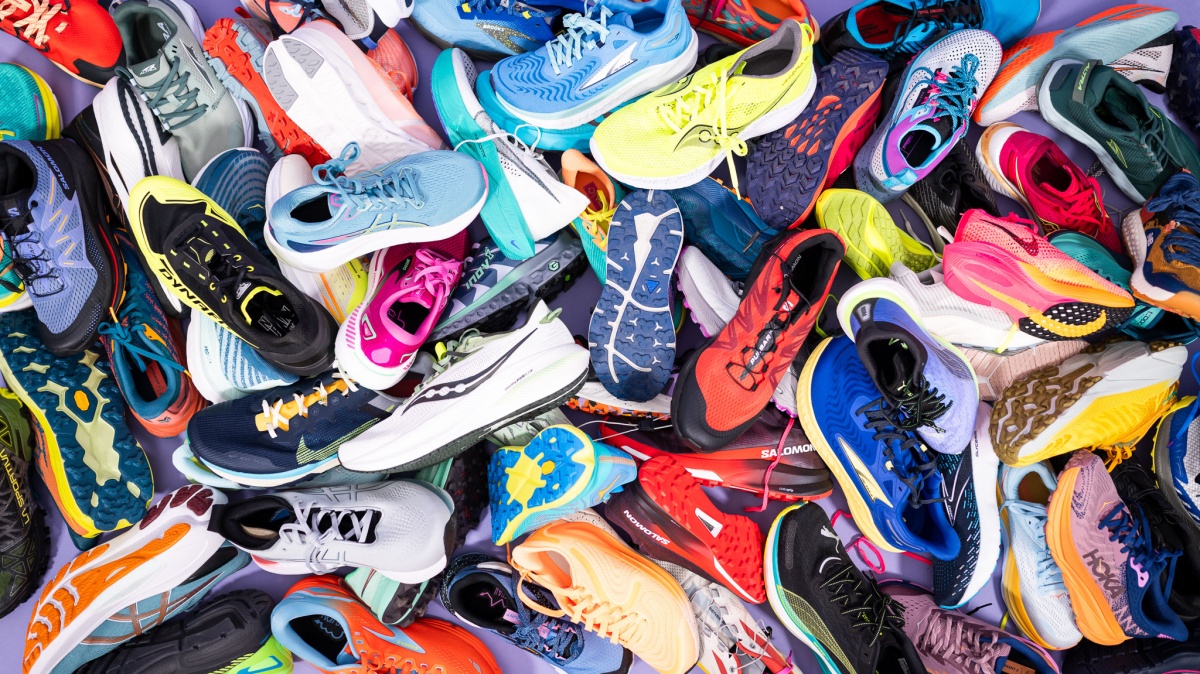The image captures a vibrant, chaotic pile of athletic sneakers in a mid-range close-up shot. The sneakers are primarily running shoes, showcasing an array of bright and diverse color schemes. Among the jumble, recognizable brands include Saucony, Hoka, Nike, Asics, and Adidas, with no two pairs matching. The shoes feature a spectrum of hues: pink, yellow, white, black, blue, green, purple, orange, gray, and various combinations of these colors. Some sneakers are upside down, while others are right side up, revealing colorful soles and laces ranging from reds and blacks to whites and blues. The image is a kaleidoscope of styles and colors, with shoes overlapping in a seemingly endless, vibrant collage.